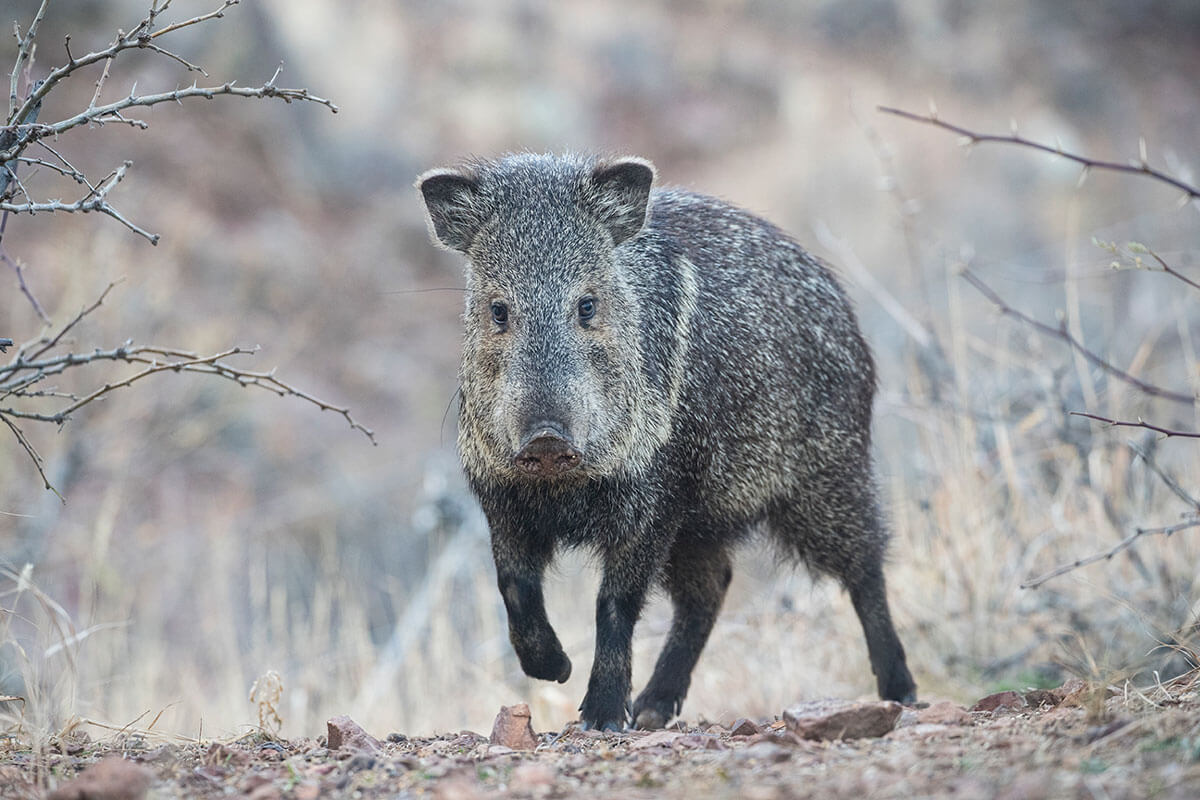This photograph captures a detailed scene of a wild pig in an outdoor setting that appears to be late winter or early spring. The ground is covered in a mix of rocks, twigs, and dead leaves, with no visible greenery. The central focus is the wild pig, which is walking towards the camera. It has a furry coat that is a speckled mix of brown, black, gray, and white. The pig has a long snout, two small ears, and black eyes, with noticeable thin whiskers. Its fur suggests it might be wearing a winter coat, well-groomed except for spiky fur between its ears. The pig’s feet are black, and its underbelly also has black fur, contrasting with tan and white speckles on its back. The background of the image is blurred, emphasizing the pig, while the surrounding area is filled with scattered twigs and small thorny shrubs, adding to the grayscale, wintry atmosphere.